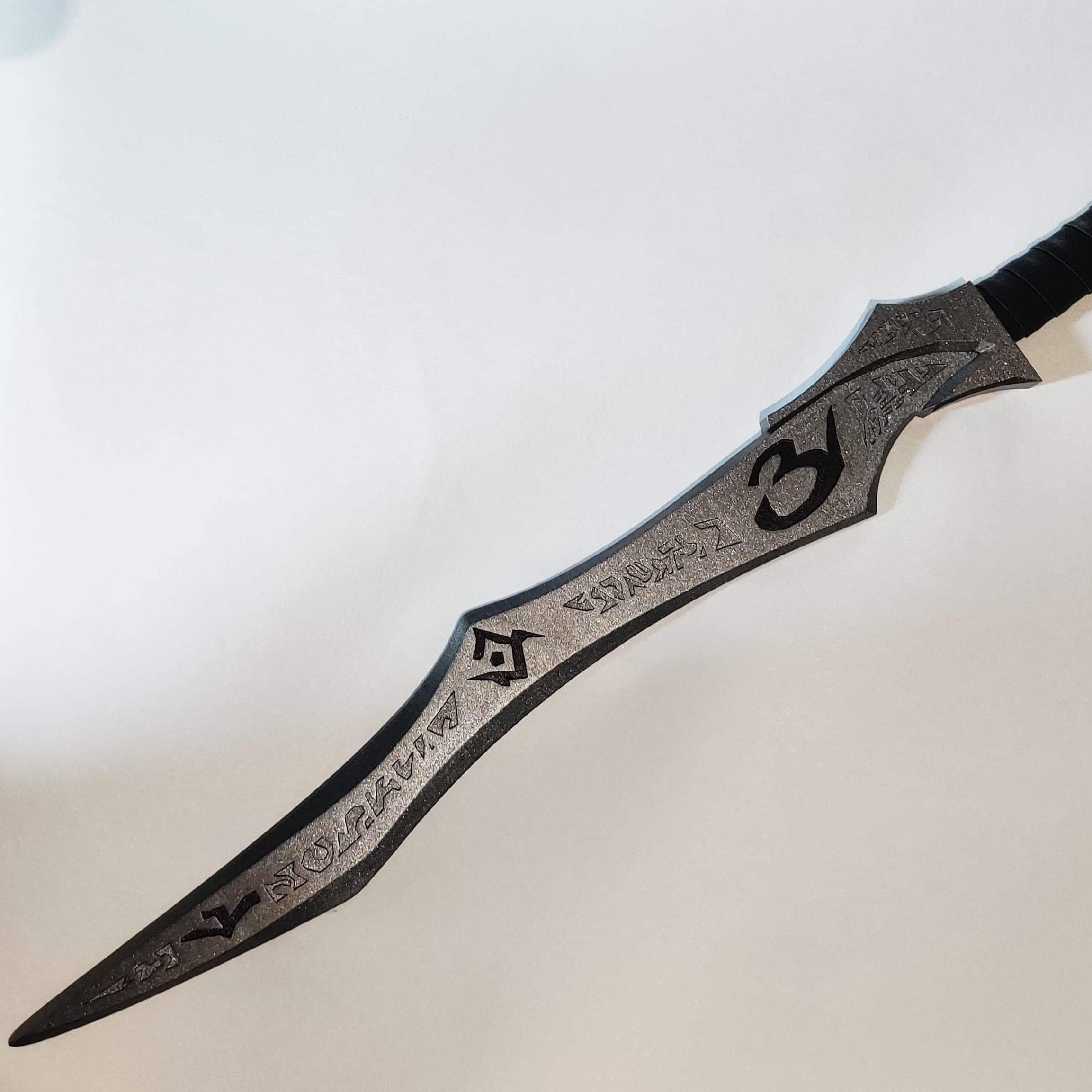The image features an abstract painting in the background, starting in the top left corner with a bit of blue that transitions into a sky blue with clouds. This blue region blends into a pinkish tan hue extending horizontally. Dominating the central part of the image, a knife lays diagonally from the upper right to the lower left. The knife has a thin, black handle, possibly wrapped in leather, situated toward the top right corner. The blade, which is silver-gray, showcases intricate designs, including Japanese or Chinese symbols. Near the handle, there is a prominent black number "3," along with other various engravings such as a diamond with a dot in the middle and a distinctive "Y" shape at the blade's far end. The blade also bears the inscription "Hakuvia" and an additional indiscernible marking. A subtle gray shadow is cast in the bottom left corner, adding depth to the otherwise minimalistic scene.